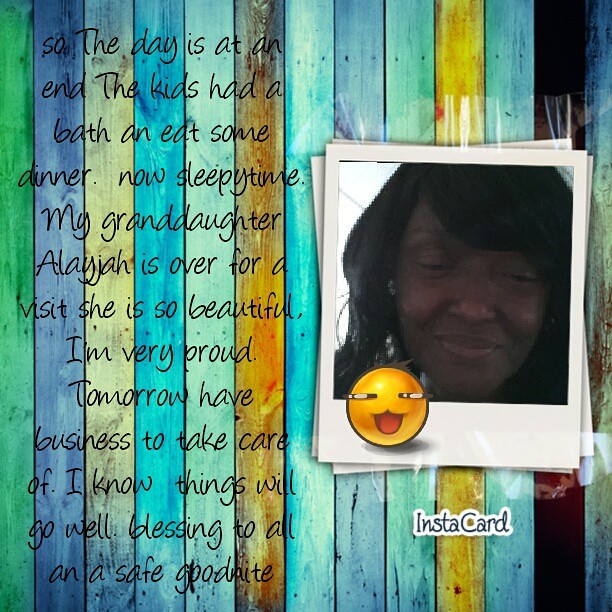This photograph captures an African-American woman, likely middle-aged or perhaps slightly older, with dark brown skin and dark brown hair. The image is styled as a Polaroid, set against a vivid backdrop of colorful wooden panels in hues of green, purple, cream, blue, turquoise, and gold. Accompanying the image is a yellow face emoji with slotted eyes and a wide-open red mouth, adding an expressive touch.

The text surrounding the image reads: "So the day is at an end. The kids had a bath and ate some dinner. Now, sleepy time. My granddaughter, Alaya, is over for a visit. She is so beautiful, and I'm very proud. Tomorrow, I have business to take care of. We know things will go well. Blessing to all, and a safe good night."

This combination of heartfelt commentary and vibrant visuals renders it a sentimental, yet lively social media post, reminiscent of those frequently shared by affectionate relatives. In the lower right corner, there's a white border with the text "Instacart" ensuring it stands out against the colorful background.